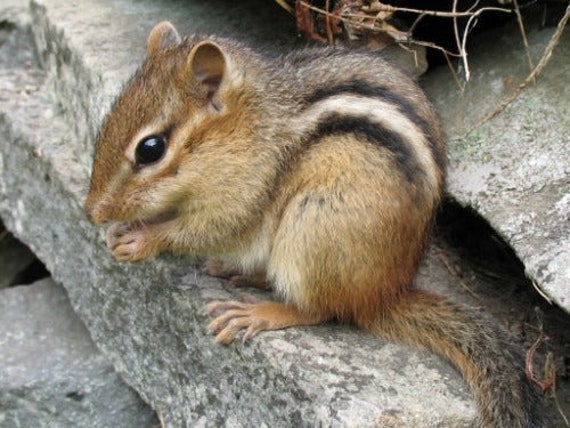This close-up photograph captures an adorable young chipmunk, often mistaken for a squirrel or "sheep-monk." The chipmunk is centrally positioned on a gray, moss-speckled rock, appearing to hold and eat a small, dark object, likely a nut or seed. The chipmunk’s body faces the camera, but its head is turned slightly to the side, showcasing its brown fur adorned with distinct black and white stripes running along its back, as well as white stripes above and below its eyes. It stands upright with its front paws lifted, bringing the food close to its mouth. The image, set in a natural environment with additional rocks and some scattered foliage, features the chipmunk's black eyes, small ears, and a curled tail. Though the photograph is a bit grainy, the realistic style emphasizes the intricate details of this charming scene in the wilderness.